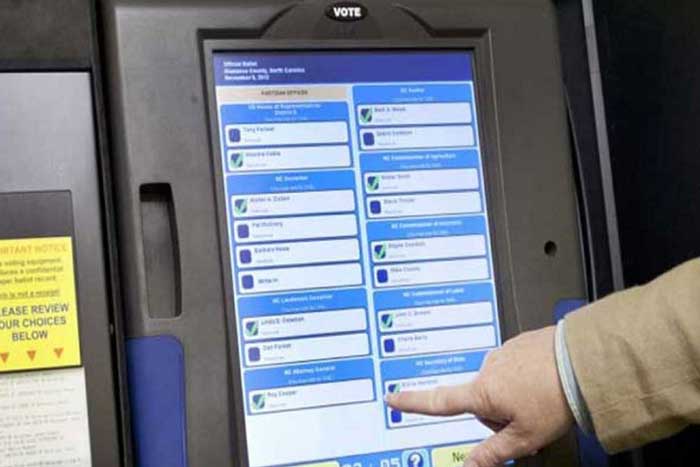The image depicts a person engaged in the act of voting at a digital voting kiosk. The setup features a touch screen direct recording electronic (DRE) system that digitally records votes. In the center of the image stands the voting machine, set at a slanted angle from left to right, with a screen displaying various candidate names alongside checkboxes. These options are categorized under light blue headings with small white text. 

A prominent hand, emerging from the bottom right corner, reaches towards the screen to make a selection. Upon doing so, a green checkmark appears next to the selected candidate. Just above the screen, a badge displaying the word "vote" in white text stands out against the black housing of the voting machine. Additionally, there is a yellow rectangular sign positioned to the left side of the display, reading "please review your choices below."

The screen and various elements are primarily bathed in shades of blue and white illumination, while an array of colors like lime green, pale yellow, gray, beige, and black add further detailing to the scene. The overall composition effectively captures the modern, user-interactive process of digital voting.